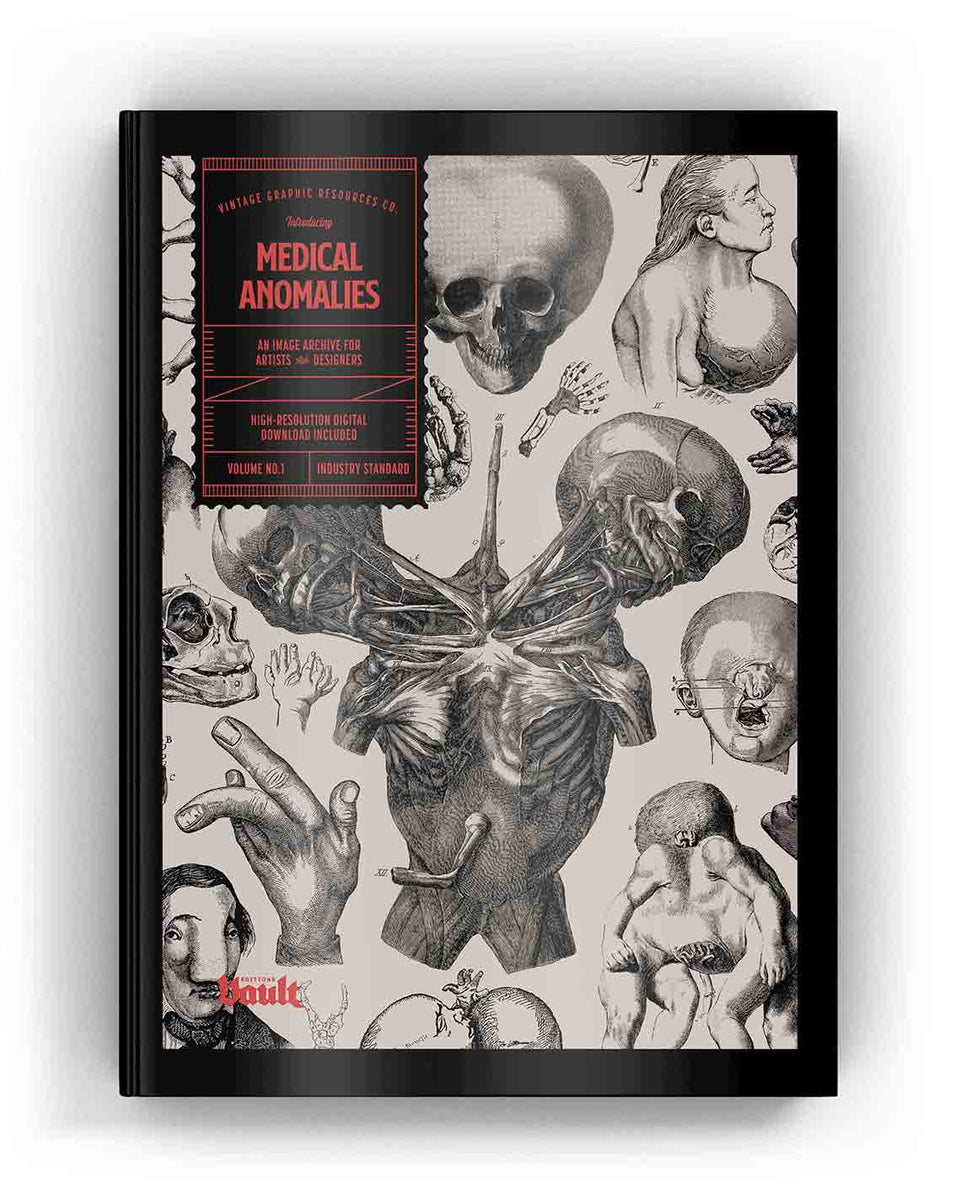The cover is predominantly black and white, featuring a central illustration that appears hand-drawn, showcasing an array of medical anomalies and deformities. The most striking image is a two-headed conjoined twin with exposed muscles and bones, flanked by a variety of other grotesque medical conditions, such as deformed hands, an enlarged breast reminiscent of a toad’s puffed throat, and skulls with various deformities. The detailed and disturbing illustrations resemble those found in vintage medical textbooks.

The title "Medical Anomalies" is prominently displayed in red font on a black background in the upper left corner, indicating that this volume serves as an image archive for artists and designers. Additional text in red declares the inclusion of a high-resolution digital download and specifies this as Volume Number One. The cover’s design incorporates a black frame with a saw blade-like edge, enhancing its archaic, almost archival feel. Smaller text within the frame, presumably the author's name and other details, is not entirely legible, though elements such as "Vintage Graphic Resources Co." and "Industry Standard" are noted. An emblem or symbol with the word "vault" also appears in the bottom left, adding to the cover’s mystique.